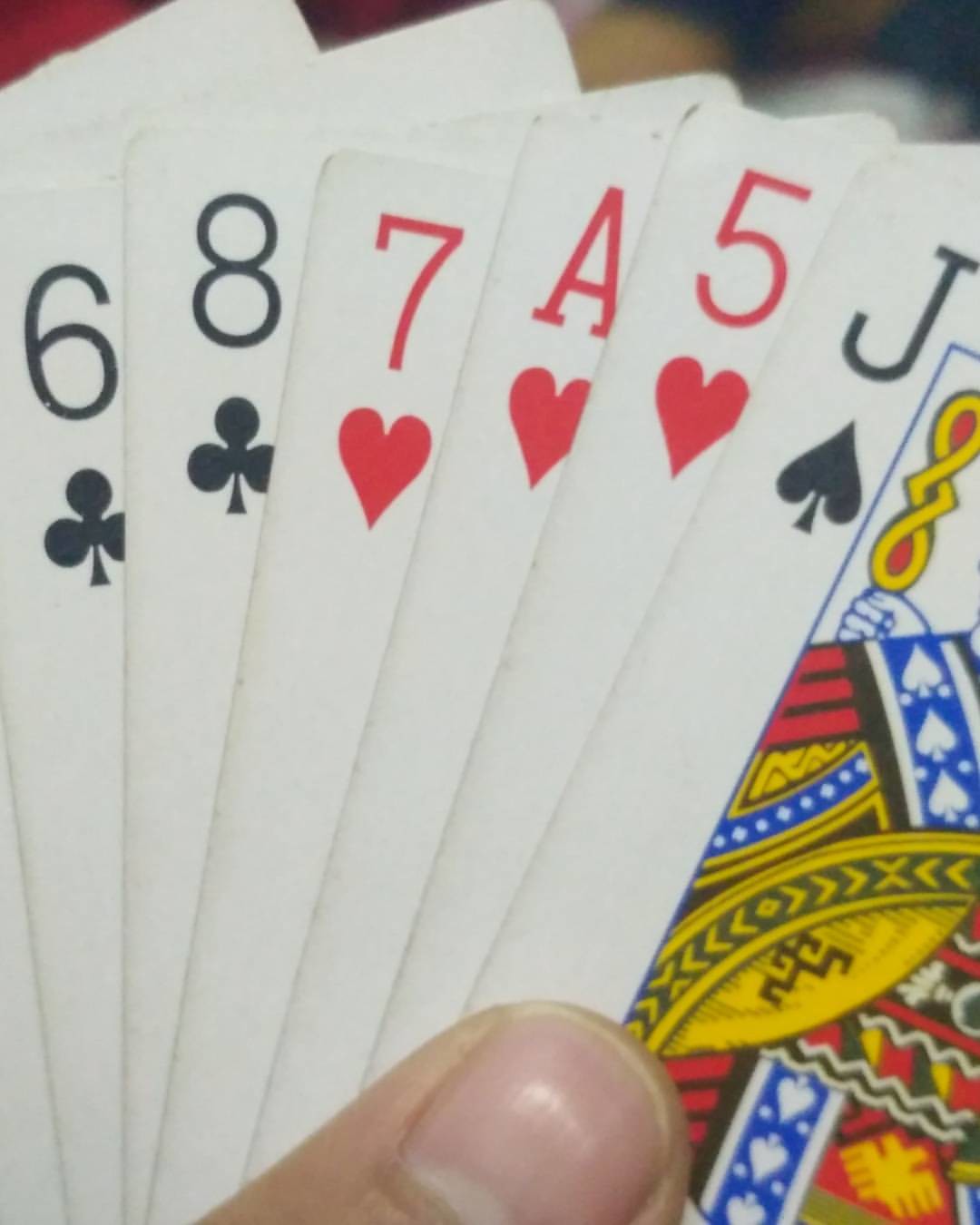In this photograph, the tip of a thumb emerges from the bottom center, stopping just below the fingernail. The thumb, which shows some skin and a bit of glare on the fingernail, is holding a fan of playing cards. The cards are as follows from right to left: prominently visible is the Jack of Spades, partly revealed. Next to it, the partial view of the Five of Hearts is visible with just the number and heart symbol. Following this, there's a glimpse of the Ace of Hearts peeking from the side, and then the Seven of Hearts. Further to the left are parts of the Eight of Clubs and the Six of Clubs. The background features a blurred red hue to the left, transitioning into black, with hints of yellow and white blending together.